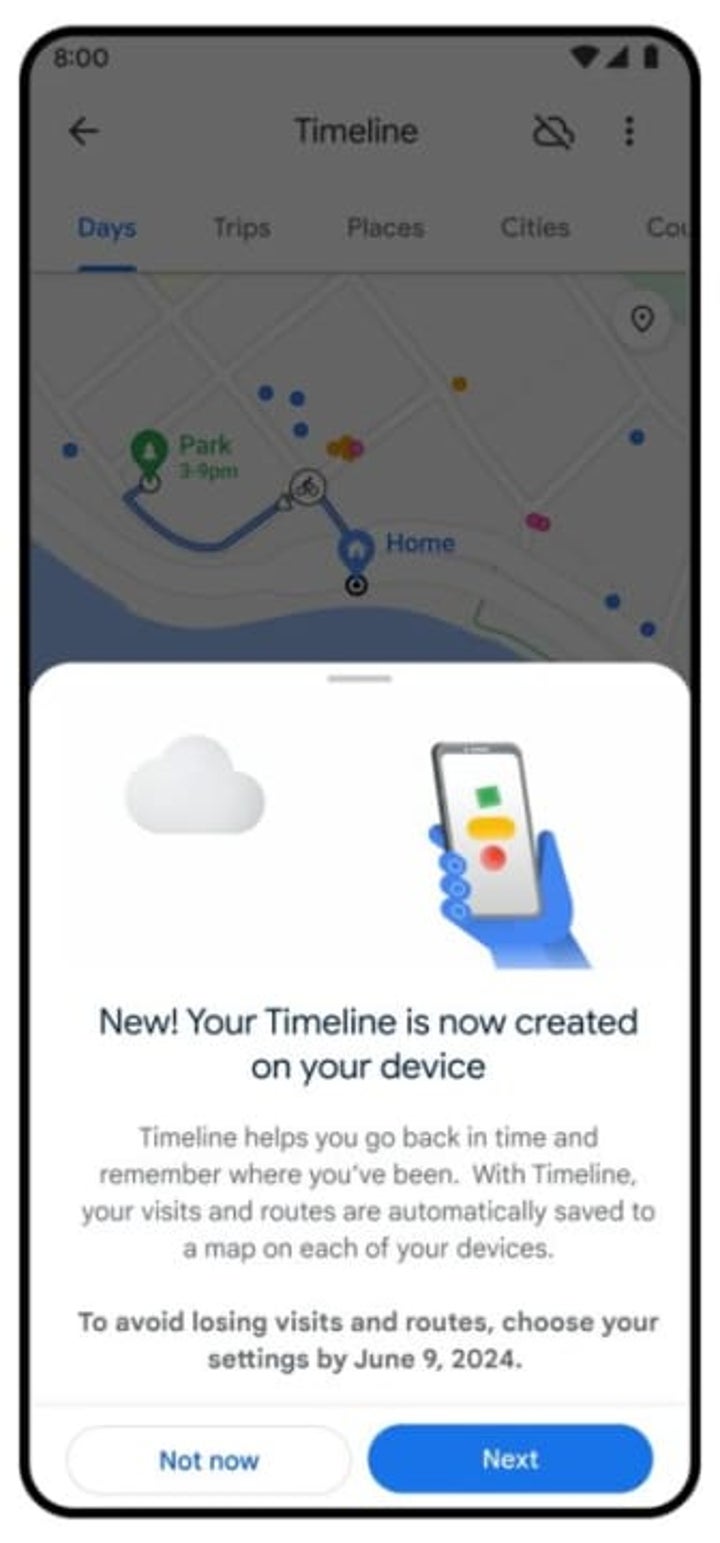The image appears to be a snapshot of a Google Maps interface. In the lower part of the image, a pop-up message is prominently displayed. Within this pop-up, on the top right, there is a blue hand holding a smartphone. The screen of the phone, shown against a white background, displays three geometric shapes: a green square, a yellow rectangle, and a red circle. To the left of the hand, the phone appears to be taking a picture of a cloud.

Beneath the hand holding the phone, the pop-up text reads: "New! Your timeline is now created on your device. Timeline helps you go back in time and remember where you've been. With Timeline, your visits and routines are automatically saved to a map on each of your devices." Following this, a darker-text notice advises, "To avoid losing visits and routines, choose your settings by June 9th, 2024."

At the very bottom of the pop-up, there are two action buttons. The button on the left, featuring blue text on a white background, says "Not now." The button on the right, with white text on a blue background, says "Next."

In the slightly faded map in the top half of the image, two locations are highlighted: one labeled "Home" with a home icon, and another labeled "Park" with an icon representing forestry.